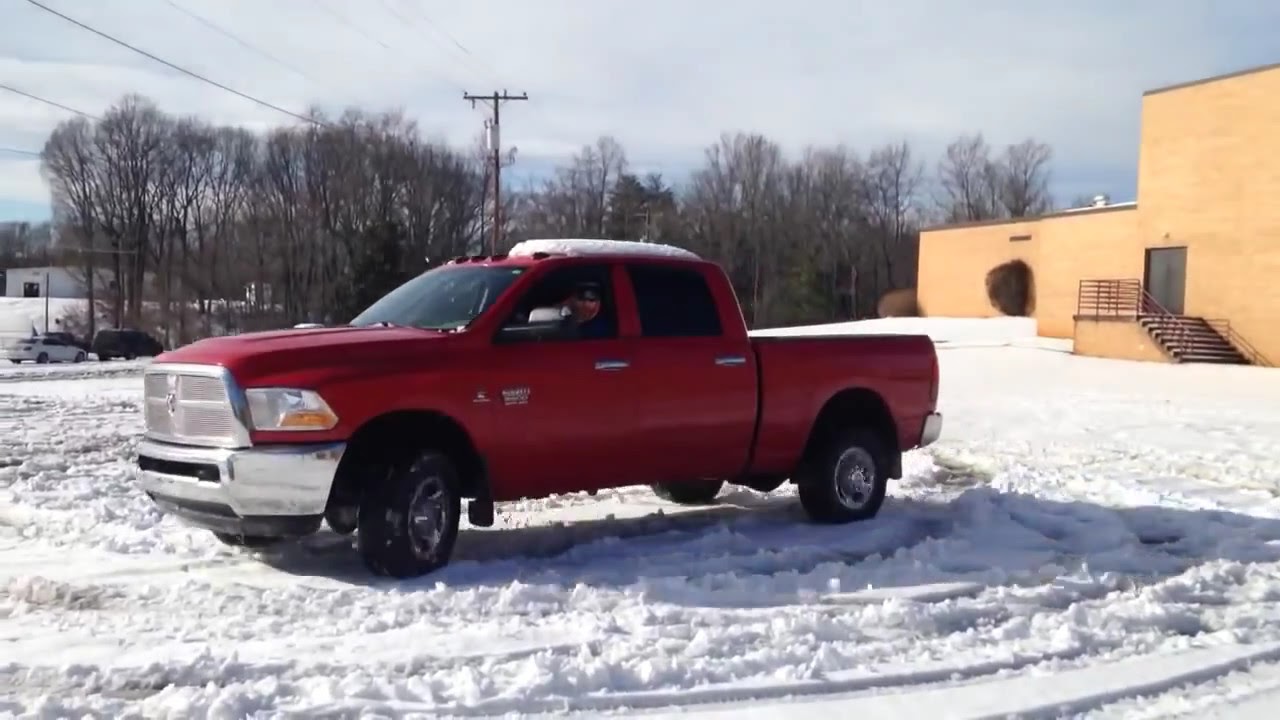In this daytime photograph set in a snow-filled area, a red four-door pickup truck with a bit of snow on its roof stands prominently in the foreground. The truck is sitting in a blanket of white snow, and visible tire tracks suggest it has been driven recently. A man with facial hair is in the driver's seat, wearing a winter coat with the hood up and a hat. His face is turned toward the viewer.

To the right of the truck is a tan-colored building with black doors and metal handrails leading up a set of stairs. In the background, barren trees with no leaves stand against a partly cloudy blue sky. Beyond these trees on the left, a white building is partially visible, accompanied by at least three vehicles—one white and two dark-colored—positioned at some distance. Additionally, a telephone pole and its utility wires can be seen near the left side of the scene.